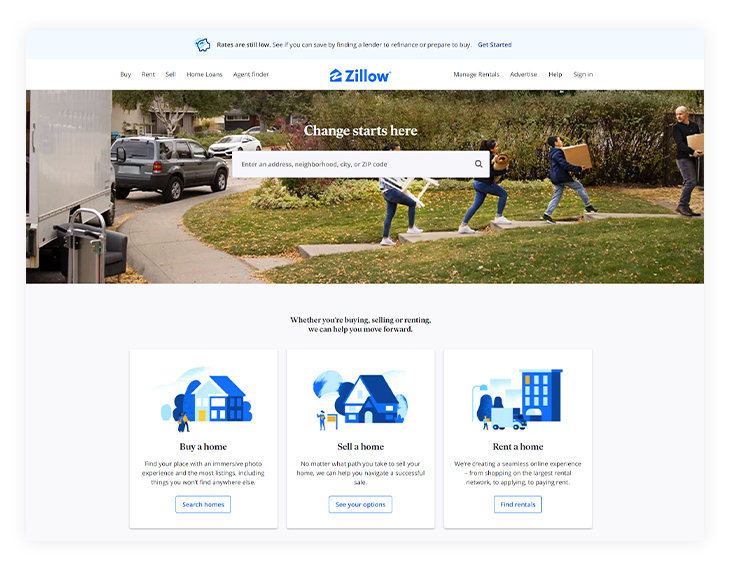The image depicts a Zillow website interface with a prominent blue Zillow logo in the center. To the left of the logo are five categories, while to the right are four categories. At the very top, there's a light blue background with a black sentence, followed by a "Get started" link in blue on the right. Underneath the Zillow logo, the tagline "Change starts here" is displayed in white text.

The background showcases an outdoor environment with a curved sidewalk, a gray SUV, and a trailer that appears to be light gray or white. The scene features a front yard divided by steps, and in the middle ground, four family members are viewed from the side carrying either a gray or cardboard box, indicating a move into a new home. Behind them, short green trees add to the suburban landscape.

Further in the background, there's a white car and part of another house, which is gray. Below the main tagline, the text reads, "Whether you're buying, selling or renting, we can help you move forward." Beneath this text are three options: "Buy a home," "Sell a home," and "Rent a home," each accompanied by a blue house icon and a corresponding blue option button. This portion of the image has a light gray background, contributing to the clean and organized layout of the Zillow web page.